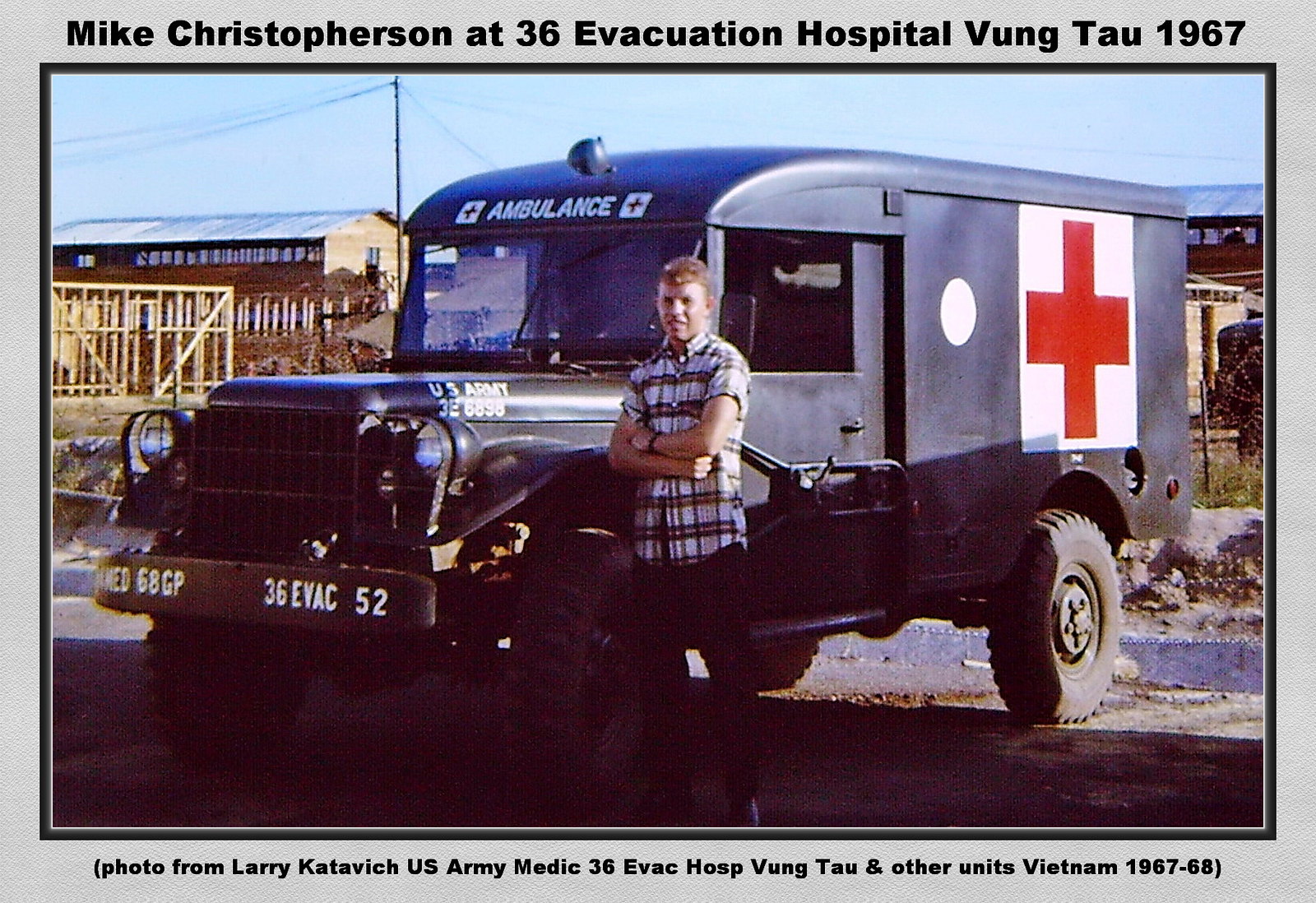This photograph, taken during the Vietnam War in 1967 and credited to Larry Katavich, U.S. Army Medic, at the 36th Evacuation Hospital, Vung Tau, features a young man named Mike Christopherson standing with his arms crossed in front of a U.S. Army ambulance. The man is dressed in a white checkered dress shirt with brown and black details, and dark pants, with the shirt sleeves rolled up. The ambulance, similar to the boxy types seen on the television series M.A.S.H., displays prominent white squares with red crosses, with "Ambulance" written on its side and the hood marking "U.S. Army 326 898." The front bumper bears the markings "6 8 GP 36 evac 5 2." In the background, wooden structures and buildings are visible, hinting at a makeshift military setup. The photo captures a moment in the hospital parking area during a tumultuous time in history.